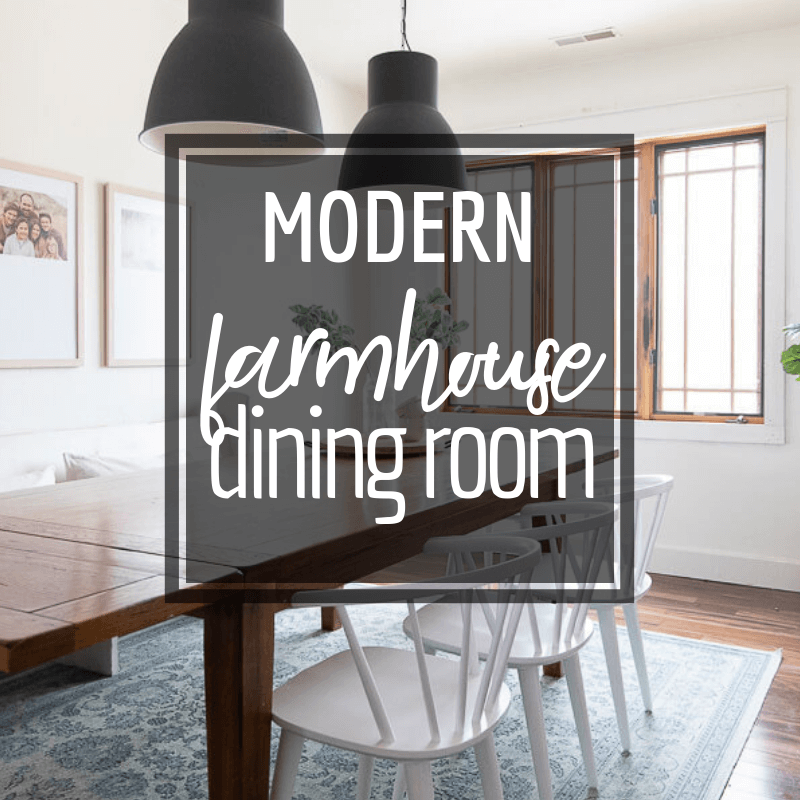This photograph, labeled "Modern Farmhouse Dining Room" in a slightly translucent black box with white print, showcases a stylish blend of modern and rustic elements. The room features white walls and a matching white ceiling, highlighting the space's clean and airy feel. Suspended from the ceiling are sleek black metal lamps with white interiors, adding a modern touch.

The focal point of the room is a medium brown wooden dining table accompanied by three white chairs, all placed atop a white rug with a subtle gray floral pattern. The rug rests on wooden flooring, which enhances the farmhouse aesthetic.

On the far wall, there are two photographs in wooden frames, possibly depicting family members. The distressed wooden window sill and paneling add to the room's rustic charm, while the window itself is divided into three parts, each subdivided into smaller rectangles by wooden muntins.

A small portion of white furniture—potentially a bench or couch—with pillows is visible on the right side of the dining room. Additionally, a few green leaves can be seen in the upper right corner, suggesting the presence of a plant just out of the frame.